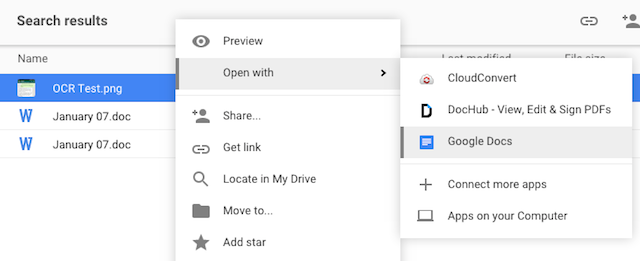A cluttered computer screen displays multiple pop-up windows and navigation options. At the top, a light gray bar with black text reads "Search results," offering various clickable options. Below this, a highlighted file named "OCRtest.png" appears in white with a blue background. Further down, there are multiple icons with a blue "W," denoting Microsoft Word documents like "January 07.doc," listed twice.

On the open tab section, a white tab displays the options "Preview" in dark gray and "Open with," both explicitly visible. The interface also includes options such as "Share…" and "Get link," followed by "Locate my drive," "Move to…," and "Add star."

The user has clicked on the "Open with" tab, revealing additional choices: "Cloud Convert," listed first in black text, followed by "Doc Hub - View, Edit, & Sign PDFs." The selected option, "Google Docs," is highlighted in gray. Below this, there is an option to "Connect more apps" and a section titled "Apps on your computer" with a laptop icon.